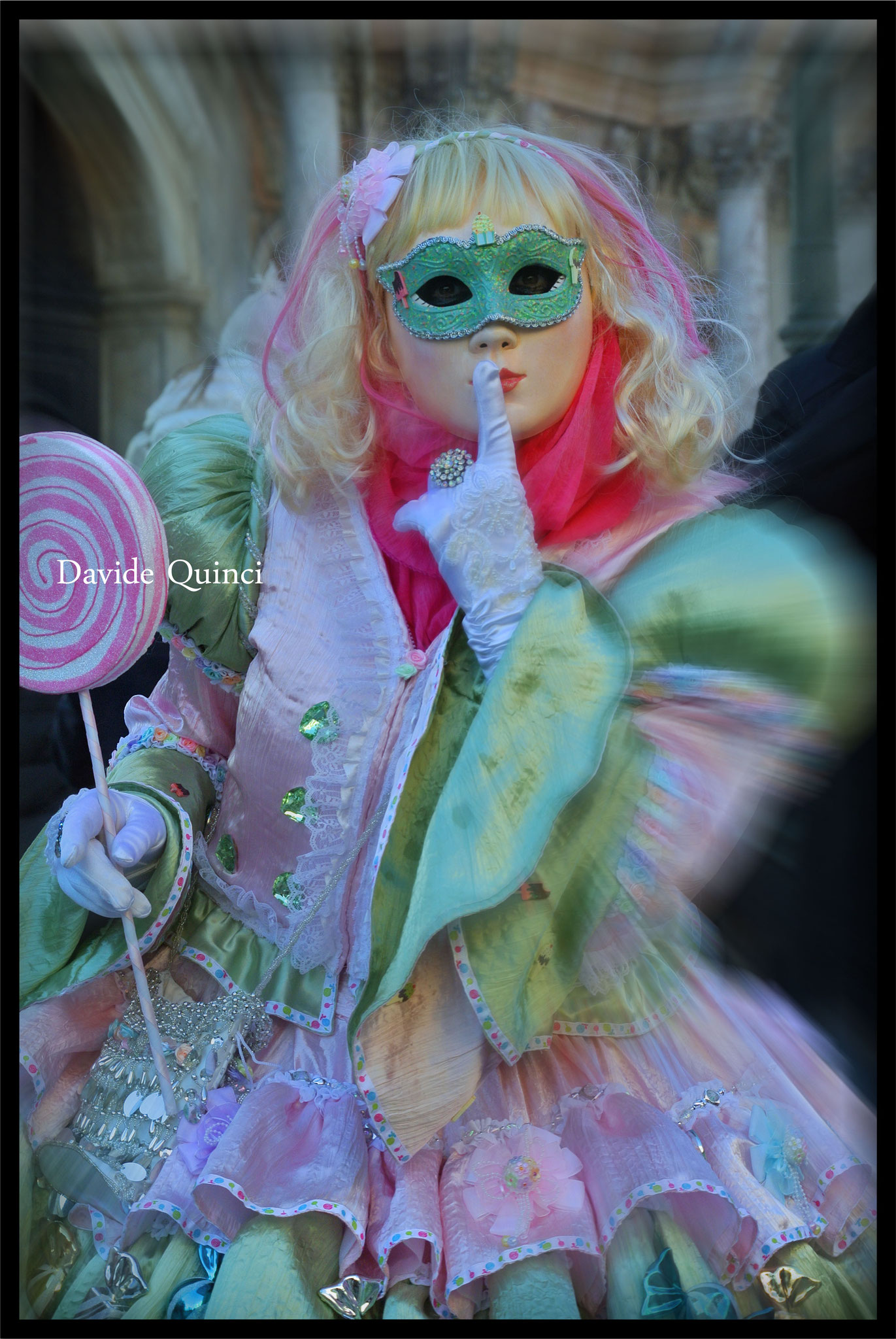The photo features a woman with light-colored skin and bright red lips. She has short, curly platinum blonde hair with straight bangs and pink streaks. She is wearing a green mask that obscures her eyes, which appear almost black, like sunglasses. Her elaborate costume is reminiscent of a 19th-century style, featuring a puffy, billowy green dress with pink highlights, including pink ruffles on the skirt and a pink vest. The dress is adorned with various jewels or sequins in multiple areas, and she dons light purple gloves on both hands. The woman is making a "shh" gesture with her left hand, pressing her gloved index finger, which has a ring on it, to her lips. In her right hand, she holds a large pink and white swirled lollipop.